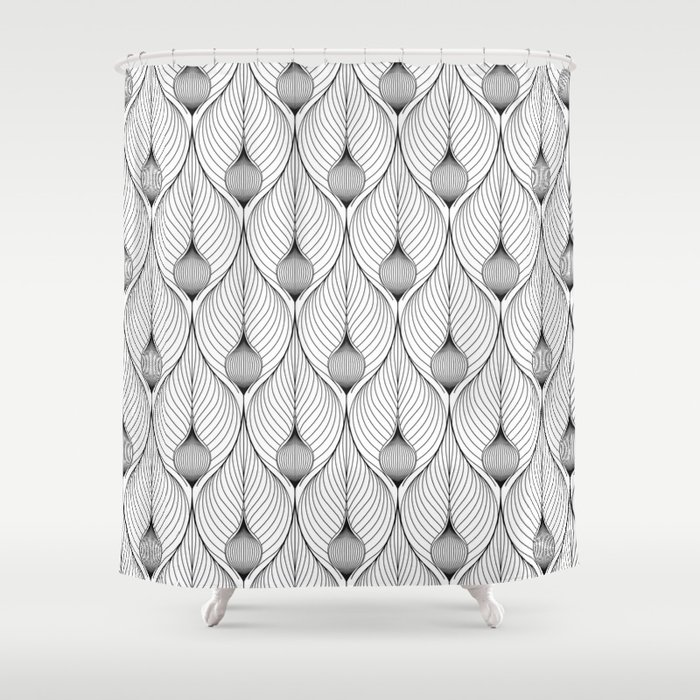The image depicts a monochrome scene with a vintage clawfoot bathtub, partially obscured by a detailed shower curtain. The curtain, suspended from a white, circular shower rail with evenly spaced silver metal hooks, features a striking black-and-white pattern reminiscent of peacock tail feathers or leaf shapes. Each motif, with vein lines running centrally, forms a smooth teardrop shape at the base, creating an elegant, repetitive design across the fabric. Below the curtain, two white iron feet of the freestanding porcelain tub peek out, suggesting the vintage style of the fixture. The backdrop of the image is stark white, casting minimal shadows and emphasizing the high contrast of the curtain and the clean lines of the tub’s legs.